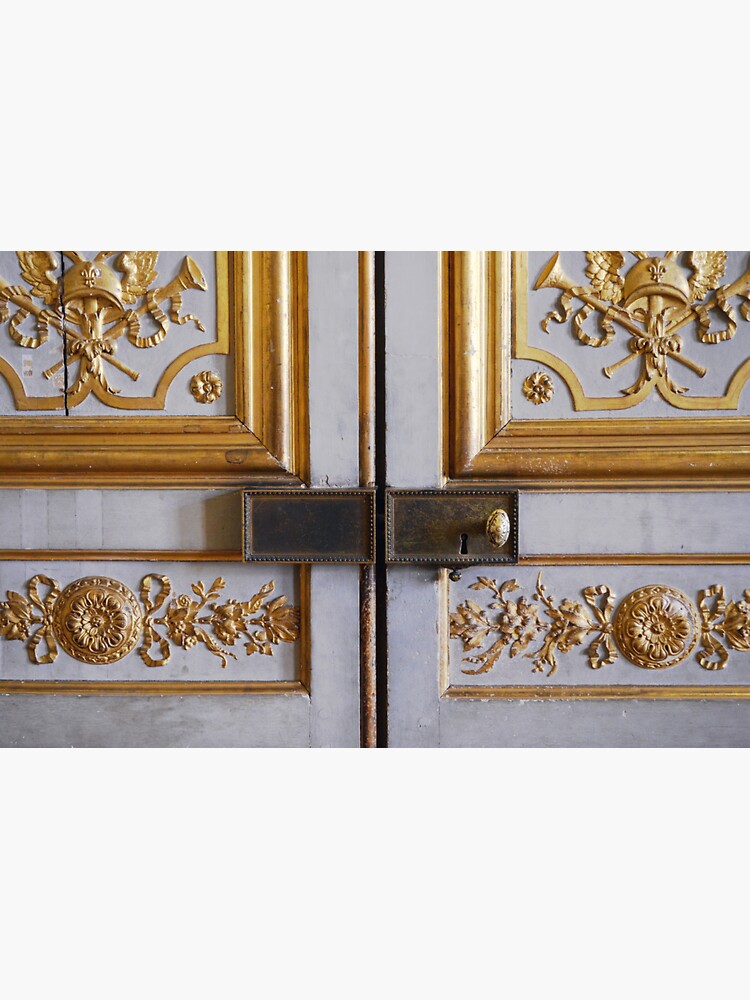In this close-up image, we see an ornate, historic double door, serving as either a doorway or a dresser/cabinet. The doors, split in the middle, are adorned with intricate design work. They are painted white, featuring faded light brownish-gold wooden paneling. Each door showcases symmetrical, elaborate gold engravings: the upper sections display interlocked trumpets with ribbon strips and what appears to be a helmet, all encased within thick gold borders. The lower sections of the doors are decorated with simpler flowery designs, also in gold. The latch in the middle is made of deep rusty brown metal and includes a gold knob on the right side, next to a keyhole. The overall intricate detailing and use of gold accents give the doors a grand, historic appearance.